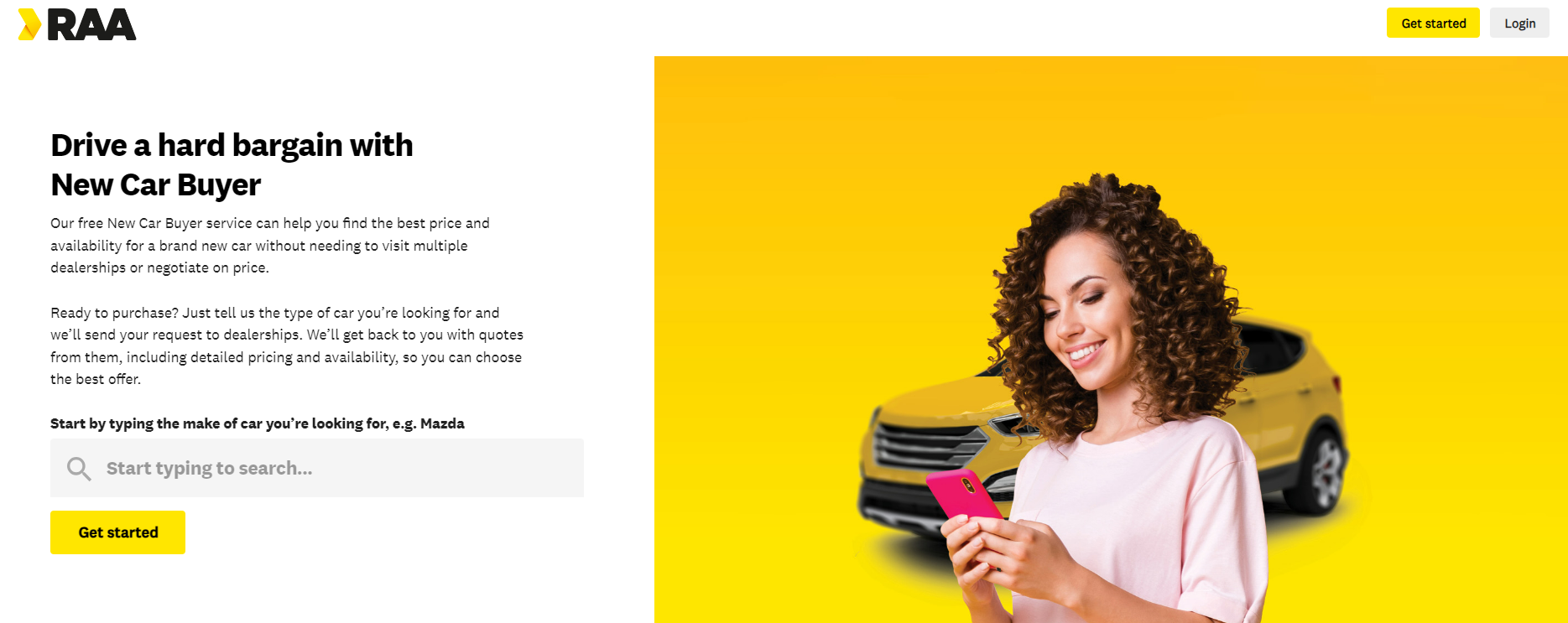In the image for RAA (Retail Automative Association), a logo featuring a leftward-pointing chevron is prominently displayed. To the left of the logo, the image is divided into two sections. The left section highlights a service tagline: "Drive a hard bargain with New Car Buyer," which refers to an online platform designed to assist users in purchasing a brand new car. The text explains that the free New Car Buyer service aids in finding the best prices and availability without the need to visit multiple dealerships or haggle over prices. 

The process is described in detail: users simply need to specify the type of car they are looking for, and their request will be sent to various dealerships. The dealerships will then respond with quotes, including detailed pricing and availability, so that users can select the best offer. 

Below the description is a gray search bar prompting users to "start by typing in the make of car you're looking for," with "Honda" given as an example. 

On the right side of the image, a cheerful woman is depicted using her phone against a bright yellow background that features a yellow car. She is smiling broadly, conveying her excitement and satisfaction with the car-buying process made easy through this service. The bottom of the image provides call-to-action buttons: “Get Started” and “Login,” inviting users to join and begin their hassle-free car shopping journey. The overall message of the image is clear: this modern service simplifies car buying much more than traditional methods.